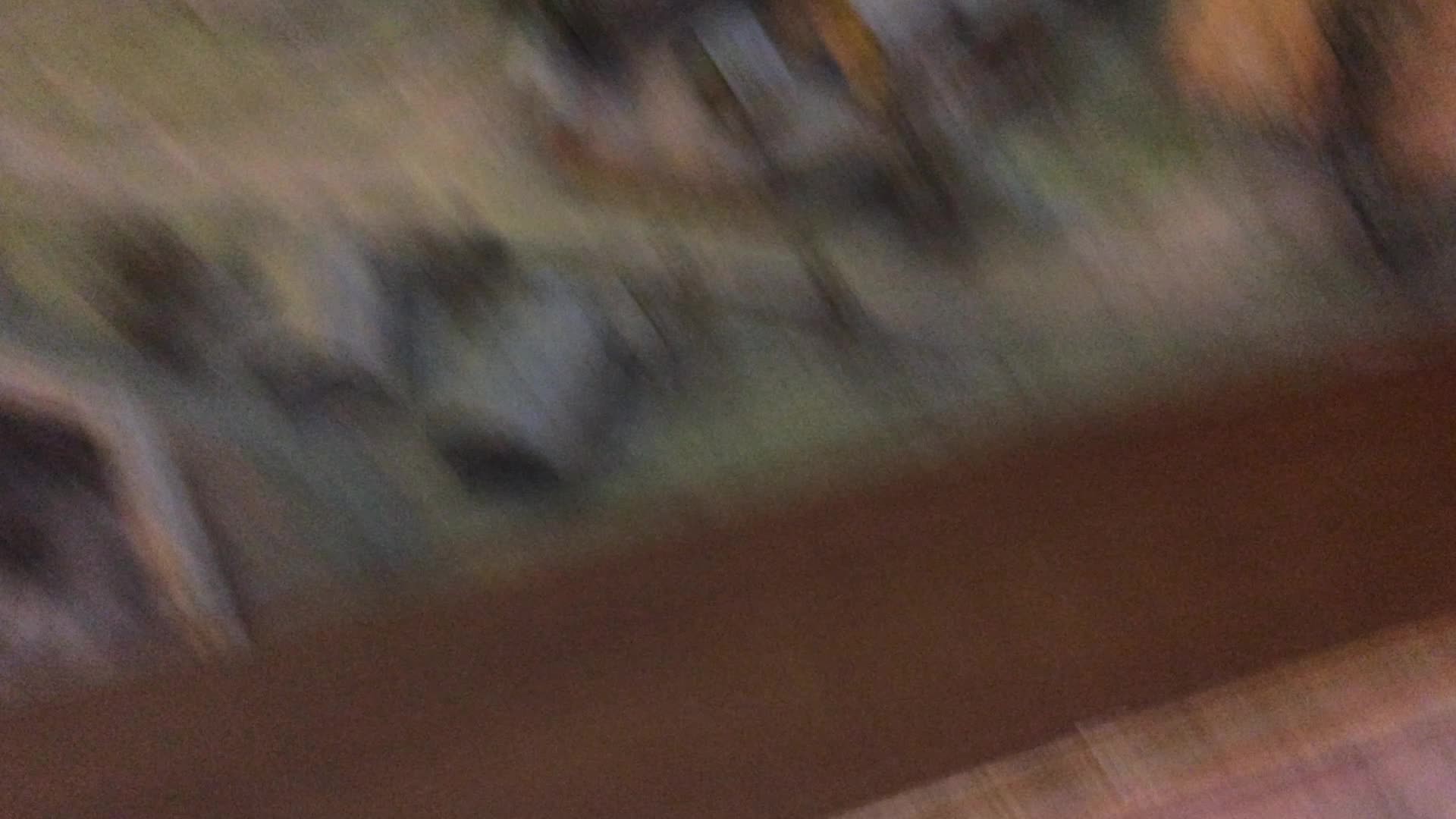A blurred photograph captures a scene with ambiguous details due to significant motion during the shutter release. The image is likely taken from indoors, possibly looking outside. A thick, deep brown rectangular shape diagonally spans the lower portion of the photo, suggesting it might be the border of a window or part of a wall. Above this, an unclear scene with green hues hints at either a piece of artwork or an outdoor landscape, resembling green grass. In the bottom left corner, there are several indistinct cylindrical, silver-colored objects. The upper right section features a bright rust-orange element, whose details are obscured by the overall blur.